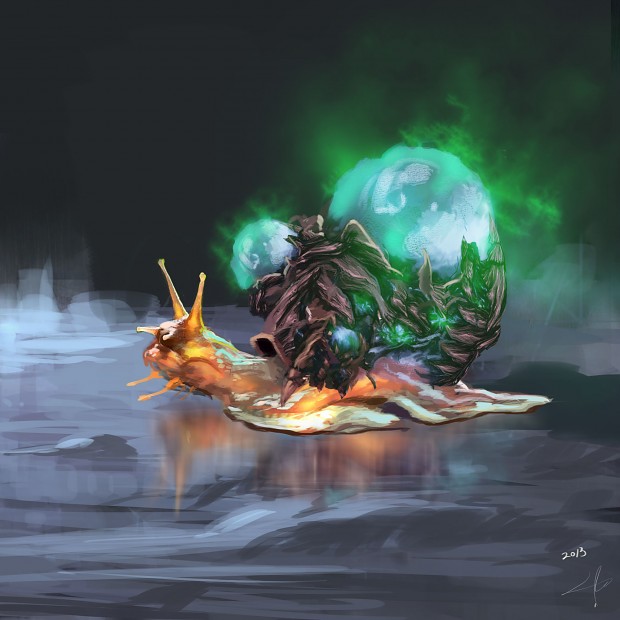This image is a striking and detailed artwork, likely hand-painted, capturing a close-up view of an unusual and fantastical snail. The central figure, which spans most of the image, is an oversized, orange-tan snail with intricate white streaks running through its body. It has two prominent antennae and additional feelers protruding from its chin, all highlighted by a faint white outline. Notably, the snail features unique botanical elements and otherworldly details—a collection of purplish-gray and green leaves adorned its back, some seeming to twinkle with tiny lights. Additionally, glowing green orbs, one large and spherical, with several smaller ones, embellish the shell situated on the snail's back, adding to its surreal appearance.

The snail is oriented towards the left side of the image, appearing to crawl on a rough, blurred surface rendered in various shades of gray and light gray. This ground covers the bottom half of the backdrop and contrasts with the smooth, dark gray to black background of the upper half, which could evoke a dimly lit room or a night sky. In the lower right corner of the image, the year "2013" and an artist's signature are visible. The overall palette includes dark gray, white, neon green, different shades of brown, black, tan, and a light green, reminiscent of northern lights, adding a mystical quality to the scene. The composition is square-shaped, contributing to the balanced aesthetic of this imaginative piece.